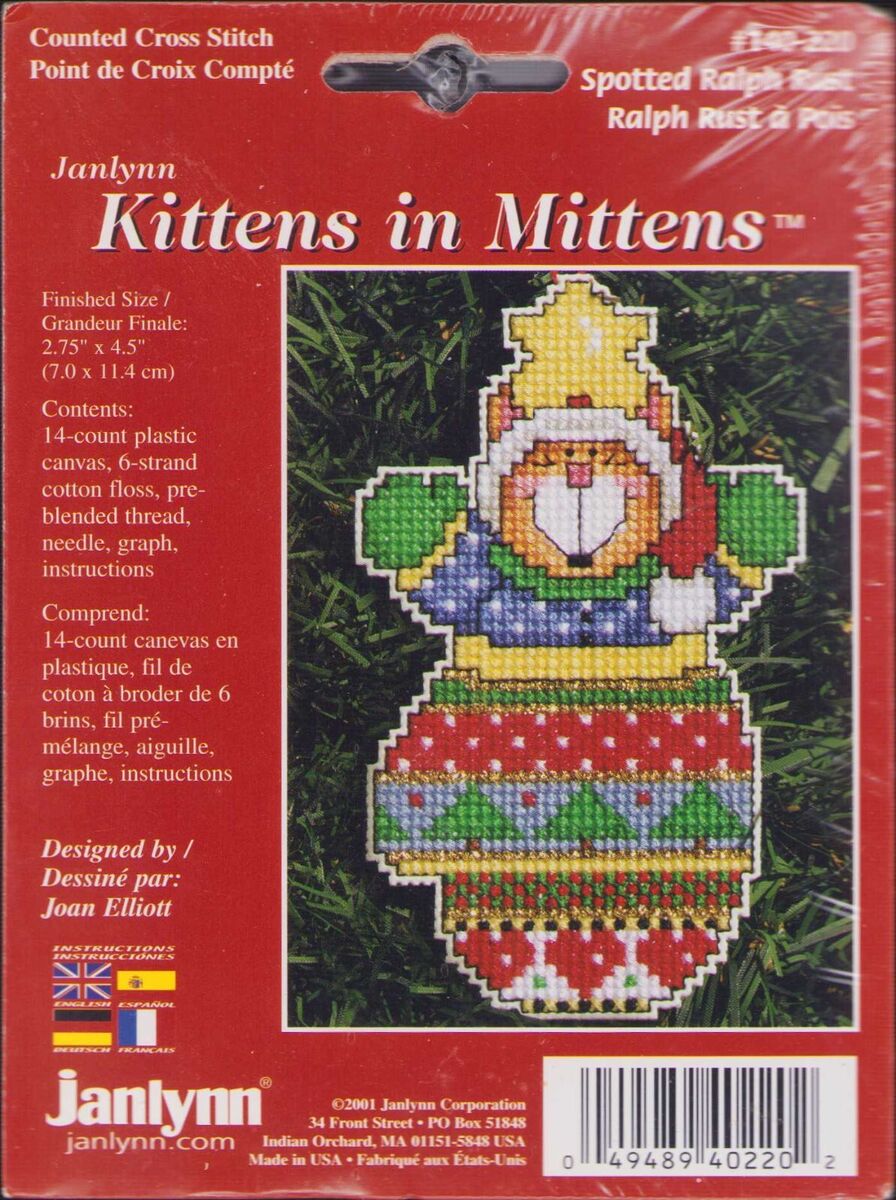This advertisement features a detailed pattern for creating a beaded Christmas-themed ornament inspired by a teddy bear. The bear, appearing as if lying on grass, is adorned in festive attire: a red St. Nicholas hat with a white trim and pompom, green mittens with yellow lining, and a blue coat dotted with white. The body is surrounded by a structured pattern of colored beads, forming shapes that evoke a Christmas tree and festive decorations in various hues such as red, green, yellow, and brown.

The bear’s face is framed by a white arc of beads, and detailed features include two dark brown trapezoidal shapes for eyes and a nose, resembling a stitched pattern. The bear's figure is accentuated with additional colorful bead patterns extending down its body, forming triangular tree-like shapes, a mix of vertical green triangles, and different colored layers toward the bottom. The background includes yellow and brown horizontal lines, and the feet are highlighted with red and white beading.

At the top of the image, the text reads "Counted Cross Stitch – Point de Croix Compté" in both English and French. The package details include "Contents: 14 count plastic canvas, six-strand cotton floss, pre-blended thread, needle, graph, instructions," ensuring that all materials needed for creating this festive ornament are included. The text "JanLynn," the company name, appears alongside various symbols representing countries such as Germany, the United Kingdom, France, and another unidentified flag. The pattern is attributed to "Joan Elliott," providing a professional touch to this DIY craft kit.

At the bottom right, there's a barcode, and the website "JanLynn.com" is printed on the bottom left. The packaging background is a vivid red, enhancing the festive feel of the product.

Instructions and corporation details are in both English and French, suggesting an international market. This product, ideal for holiday crafting, is made in the USA by the Jocelyn Corporation.

This ornament pattern blends traditional Christmas imagery with a modern, pixelated, almost 8-bit style, perfect for crafting enthusiasts looking to create a unique holiday decoration.